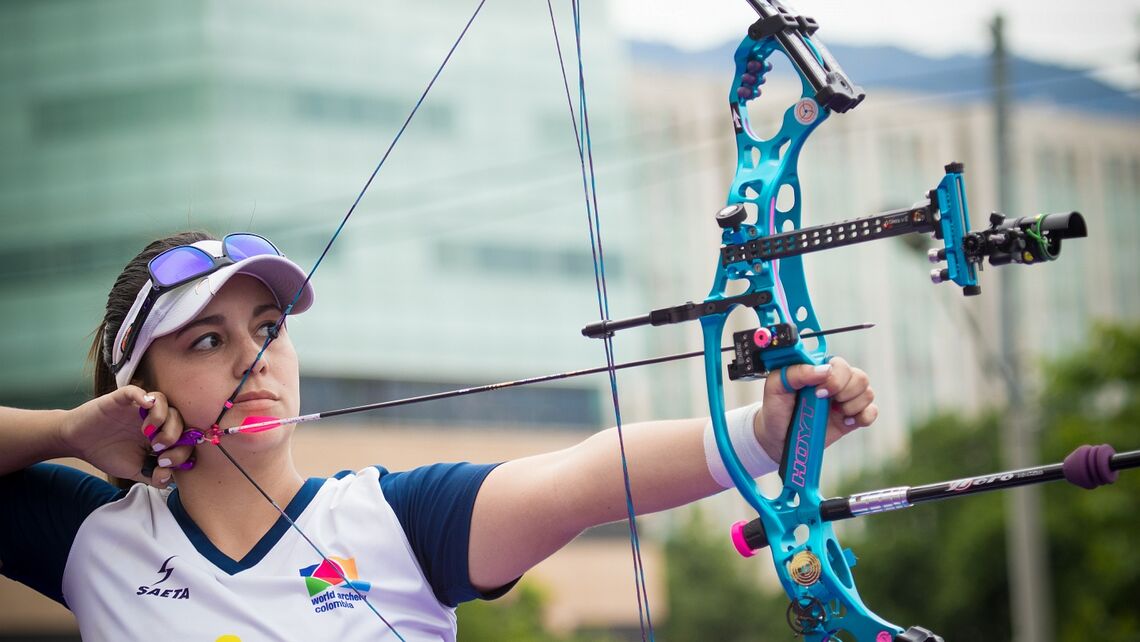In this photograph, a young woman is depicted in the midst of drawing back a vibrant pink-fletched arrow on her modern, turquoise blue compound bow. With her right arm pulling the arrow taut and her left arm steadying the bow, she appears poised and ready to release her shot. The bow itself is striking, adorned with various black tactical instruments, enhancing both its contemporary aesthetic and functionality. The woman's right hand, which grips the fletching, is positioned close to her cheek, assisted by a gripper for better precision. 

She is wearing a white and navy blue v-neck shirt, potentially from a team or organization, with the name "Sarta" prominently displayed on it. Her attire is completed with navy blue sleeves and collar trim, while a brightly colored logo adorns the left side of her shirt. Adding to her sporty look, she has a white visor with her sunglasses turned upside down perched atop it. Her brown hair is neatly pulled back into a ponytail, emphasizing her focused expression. Notably, her nails are painted white, except for her right pinky which stands out with a pink hue.

Behind her, the background subtly features muted scenery with bushes and the silhouette of a tall building, providing a serene yet urban contrast to her intense concentration. Although the location is unspecified, the clarity of her archery activity is unmistakably captured in this dynamic shot.